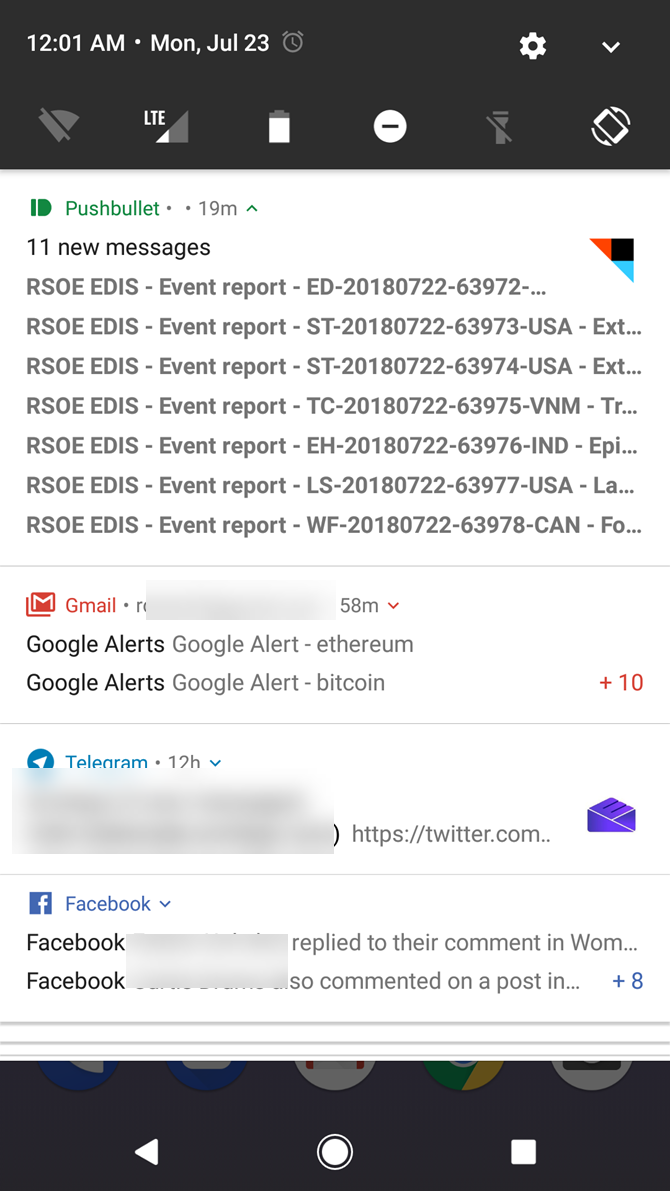Caption: 

The image depicts a screenshot from an Android phone. At the top left corner, the time is displayed as 12:01 AM, with the date indicated as Monday, July 23rd. Adjacent to this, a light gray alarm clock icon is visible. On the top right, there is a gear icon and a downward arrow icon.

Beneath this header, there are six status icons. Starting from the left, the first icon is a grayed-out Wi-Fi symbol. Next, there is a phone signal strength icon showing one bar with "LTE" labeled above it. The battery icon, which appears almost full, is approximately at 80% capacity. To the right of the battery icon is a circle with a dash inside, followed by a grayed-out flashlight icon. The last icon in this row is a phone depicted at a diagonal angle.

In the middle left of the image, the text "Pushbullet" is displayed with "19M" to the right of it. Below this line, it shows "11 new messages," followed by "R-S-O-E-D-I-S event report" repeated multiple times. Further down, applications are listed sequentially: "Gmail," "Telegram," and "Facebook" in the middle of the image.